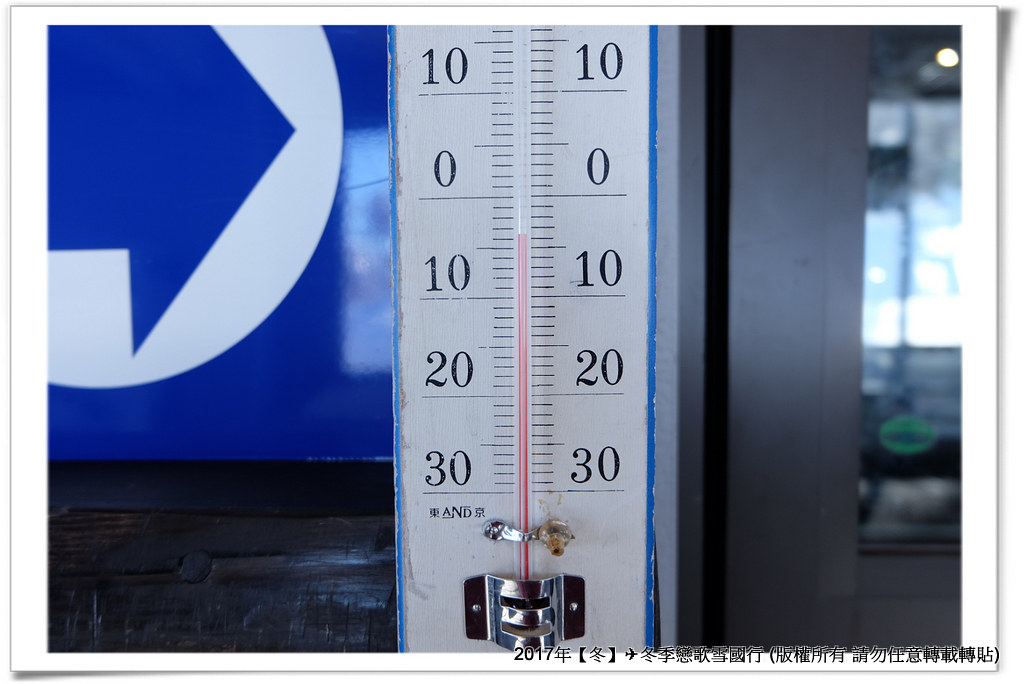The image features a detailed close-up of a white thermometer with blue trim, prominently displaying a metal clasp securing it at the bottom, and another clasp slightly above it. The base of the thermometer reads "2017." The thermometer scale ranges from -30 degrees to unknown positive temperature, marked in increments with larger lines denoting every 5 degrees and smaller lines for each degree. Currently, the temperature is indicated as approximately -3 degrees by a red line within a glass tube.

Behind the thermometer, there is a blue sign featuring a white arrow circle, directing to the right, attached to a wooden post. The background reveals a series of Chinese characters, their exact meaning unknown. The setting appears to be inside a building, as suggested by the glass wall and door visible to the right side of the image, leading to the outside.